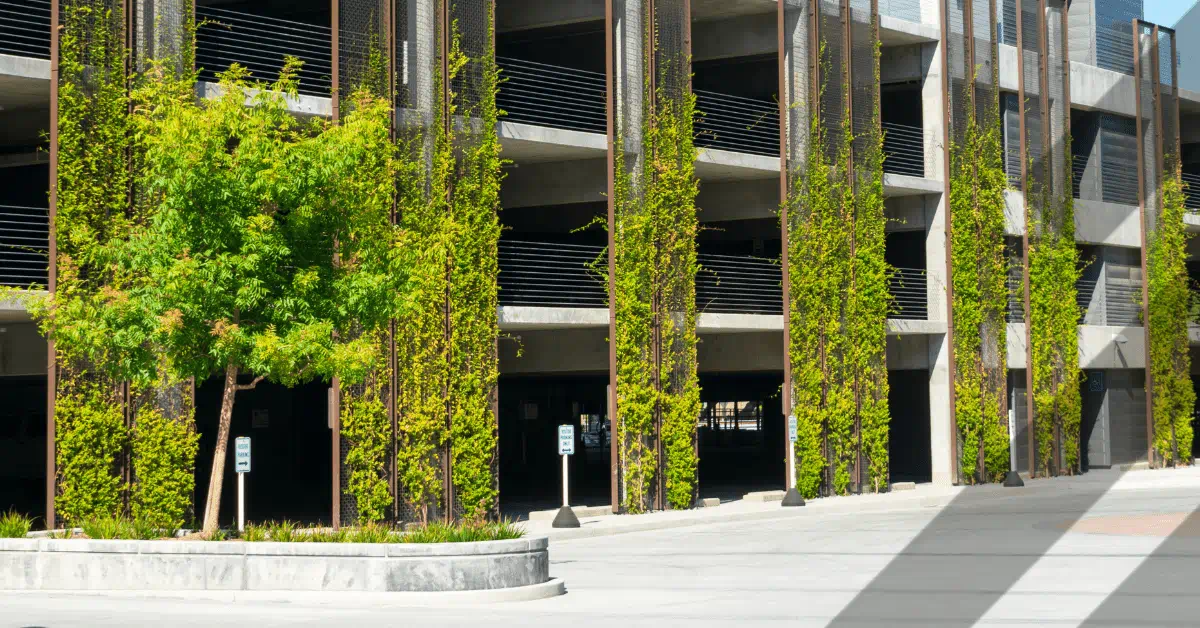This photograph captures a large, light-gray structure that appears to be either an office building or a parking garage, characterized by its multi-level design—most visibly three floors. Surrounding each level of the building is a protective fencing, while brown poles or trellises adorned with lush, green ivy run vertically from the ground to the top. The ivy climbs the poles intricately, adding a touch of nature to the otherwise industrial setting. In the foreground, there is a small tree with a slender trunk, and a cement plaza stretches before the building. In the distance, the sky is blue, and various street signs, including those indicating no parking, are noticeable along the building's periphery. The street in front of the structure is clean and shows no cars parked within the garage, revealing open spaces inside.